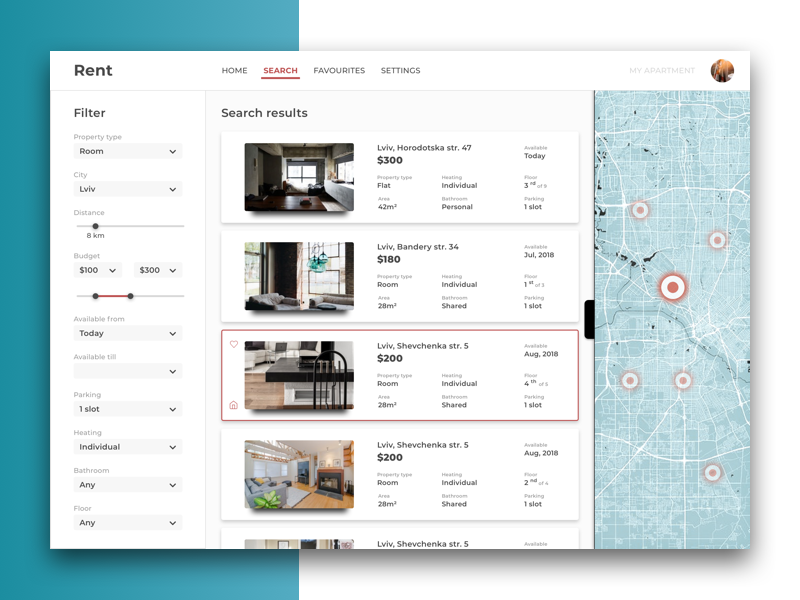This image depicts a browser window for the company Rent. In the top left corner of the browser, the company's logo, "Rent," is prominently displayed. The middle of the browser header features tabs labeled "Home," "Search," "Favorite," and "Settings." The "Search" tab is highlighted in red and is underlined, indicating it is currently active. To the far right of this row, there are icons for "Profile Pic" and "My Apartment."

Moving to the body of the webpage, on the far left side, there is a comprehensive filter section to tailor the search results. The filters include categories for Property Type, City, Distance (adjustable via a bar or slider), Budget, Parking, Heating, Bathroom, and Floor options.

The main content area, centrally located on the page, is titled "Search Results" and displays four different properties. The third property is highlighted with a red box. This listing is for "Liv Shevchenko STR.5," priced at $200. To the left of this listing, there is an image showing the apartment’s kitchen, countertop, and living room. Additional details provided for this property include:
- Property Type: Room
- Area: Approximately 28 square meters
- Heating: Individual
- Bathroom: Shared
- Parking: One slot
- Floor: Fourth out of five floors
- Availability: August 2018

To the right of the main content, there is a large, vertically oriented map with red markers indicating the locations of different properties. The map filter is set to blue. At the center edge of the left side of the map, there is a black tab.